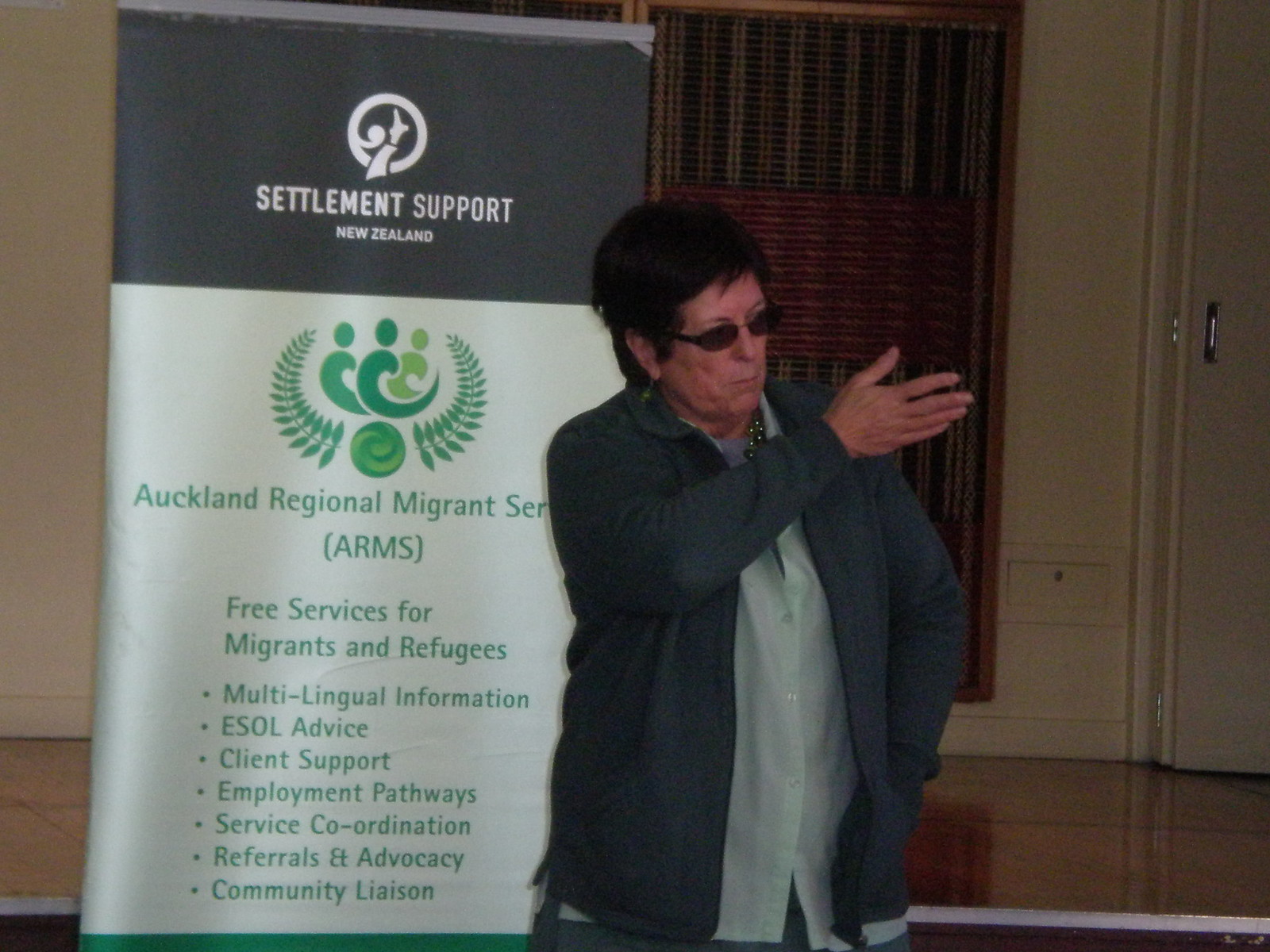In the image, an older woman, likely in her 50s or 60s, is captured in an action shot while giving a presentation. She stands near the stage of a conference hall or auditorium, gesturing with her right arm raised across her chest towards her shoulder while her other hand rests in her pocket. She is dressed in a blue overcoat over a white shirt, adorned with beads around her neck, and wearing black glasses or sunglasses.

To her left, a pop-up banner with a black top and white bottom features prominently. At the top, it reads "Settlement Support New Zealand" in bold letters. Below this, a green logo resembling a wreath with three person-like shapes is visible. The text beside the logo includes "Auckland Regional Migrant Services" and its acronym, "ARMS." The banner lists the services provided: "Free Services for Migrants and Refugees, Multilingual Information, ESOL Advice, Client Support, Employment Pathways, Service Coordination, Referrals and Advocacy, Community Liaison." The setting suggests a formal event focused on offering support to migrants and refugees.